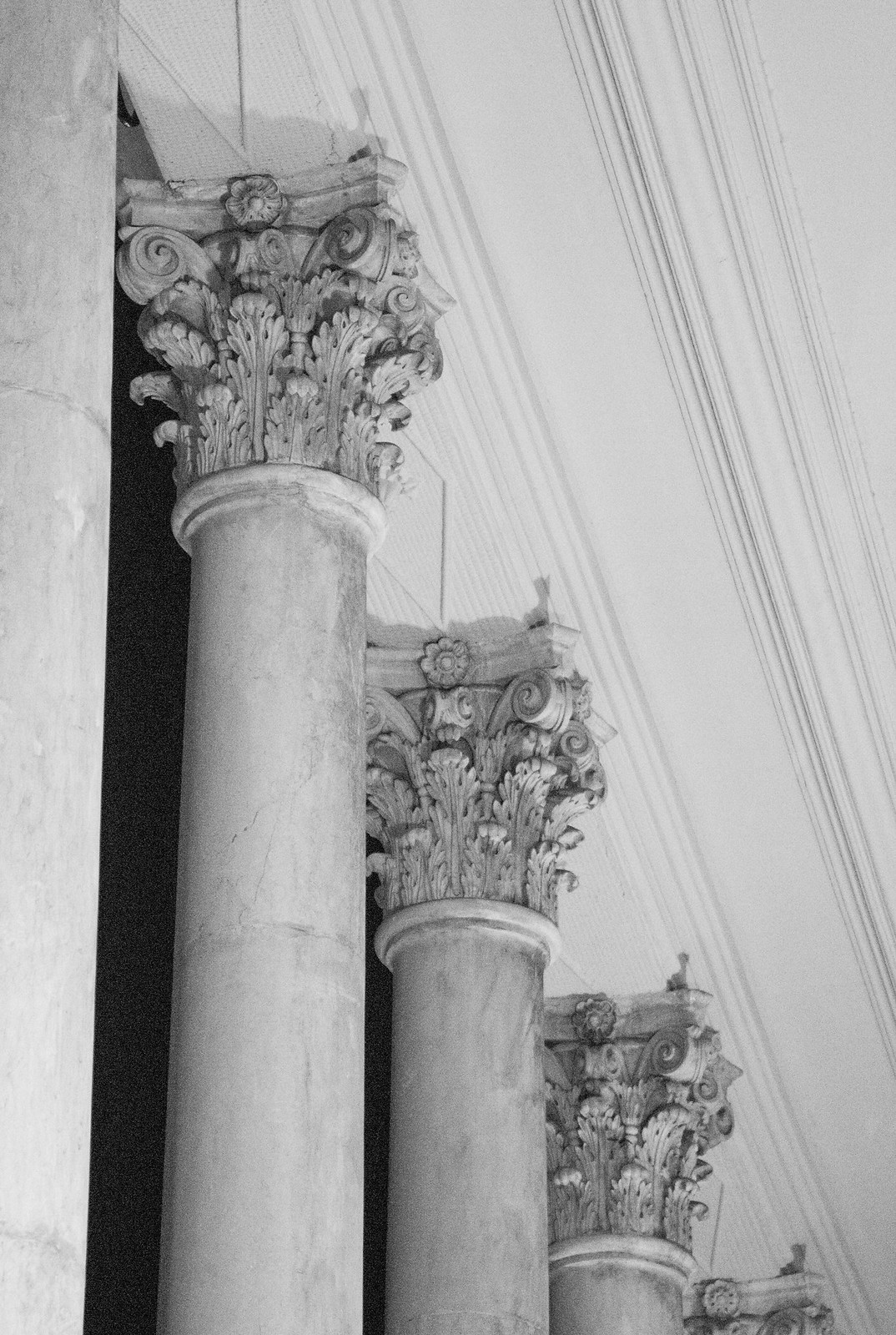The black and white image depicts an interior section of an old building, showcasing five intricately detailed columns in a row. These columns, resembling white marble, reach up to touch a ceiling that shares the same color scheme. At the top of each pillar, there are elaborate carvings of flowers and curling leaves, exuding a classical architectural style reminiscent of Roman or Greek influences. The ceiling itself also features sophisticated, old-school carvings, adding to the historical ambiance of the structure.